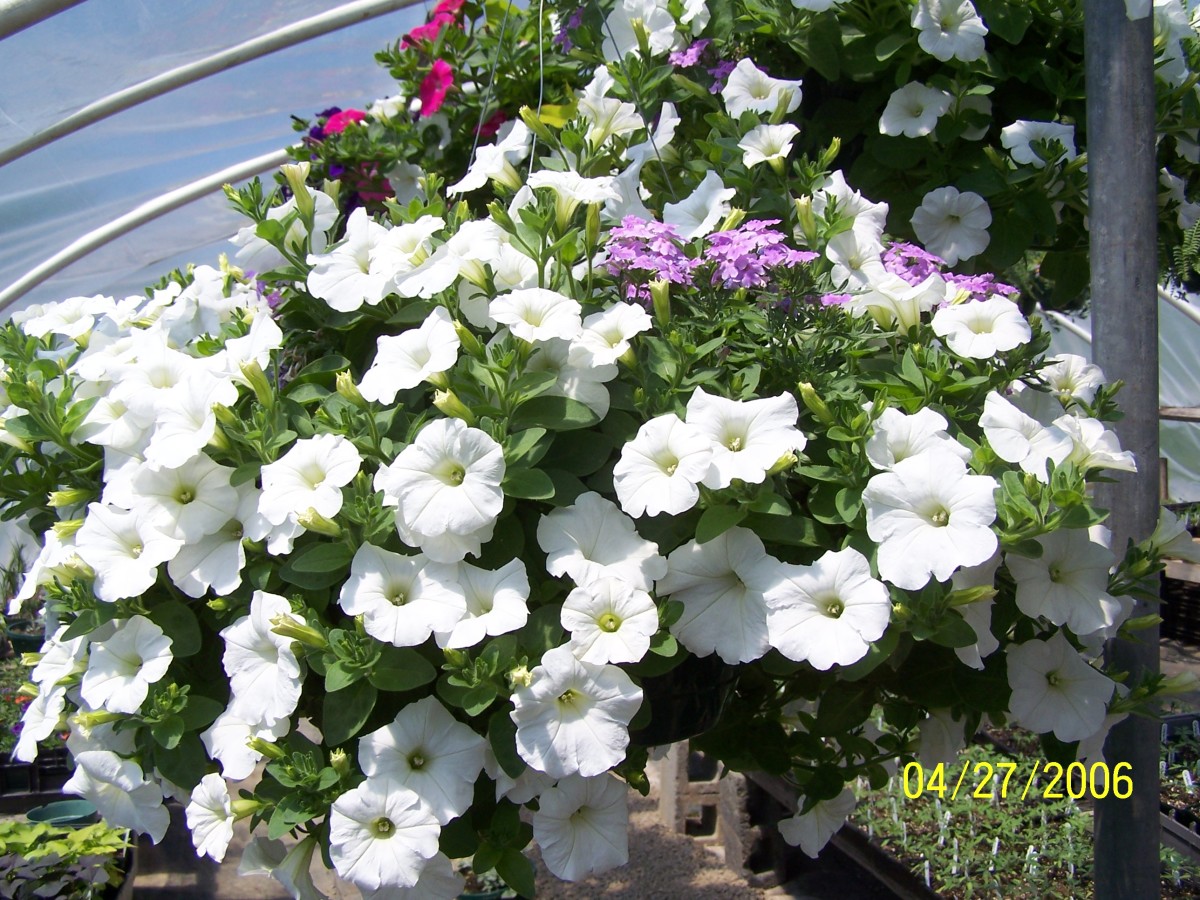The image is a horizontal rectangular photograph featuring a vibrant close-up of flowers, primarily white petunias with yellow centers, set in what appears to be an outdoor urban environment, possibly in front of a store along a street. The petunias dominate the foreground, accompanied by purple, pink, and red blossoms, the latter mostly scattered in the background. The flowers are housed in a planter attached to a metal pole. In the upper left corner of the image, there are silver railings and what seems to be a street or possibly streetcar tracks, suggesting an urban setting. Behind the railings, there's a blue and tan background that might be the sky or water. Additionally, there are gray cinder blocks below holding up shelving, indicating that the flowers could be displayed in a hoop-style greenhouse, as metal hoops are visible curving above the plants. The ground consists of gravel or sand. A date stamp in the bottom right corner, in yellow text, reads "04-27-2006."